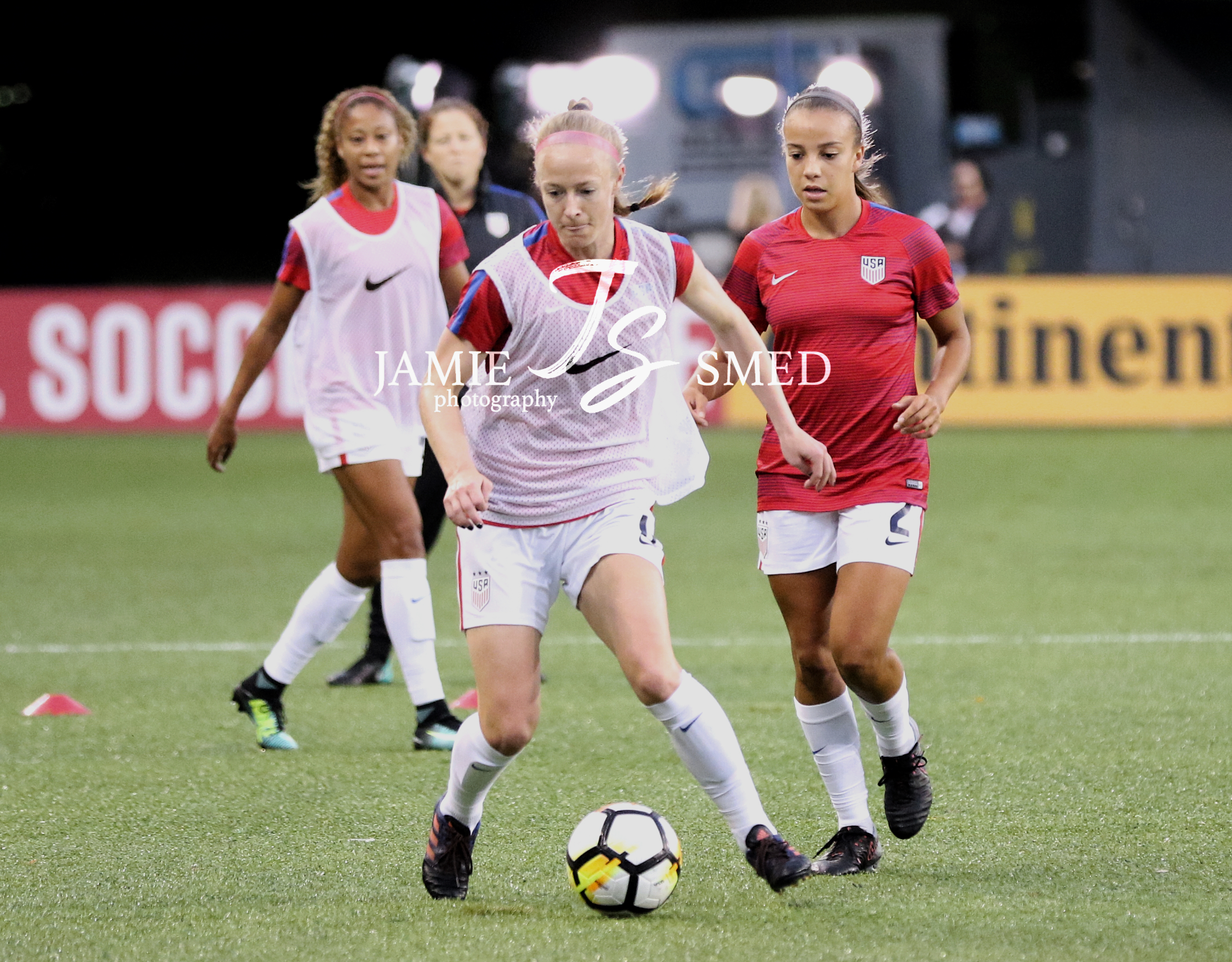This image captures an intense moment in the middle of a high school soccer game between two teams. In the foreground, a girl from the opposing team, wearing a red shirt, white shorts, white knee-high socks, and black cleats, is controlling the ball with her legs. Closest to her stands a girl from the home team, identifiable by her distinct white Nike tank top over a red T-shirt, white shorts, white socks, and black cleats. She has blonde hair pulled back in a braid and is focused on reclaiming the ball. Another teammate, also in a white top with a Nike logo over a red T-shirt, is visible nearby. In the background, a referee in a blue shirt is overseeing the game. The sidelines feature a brown background with partially visible signage that reads "S.O.C.C...." on the left and the letters "I-N-E-N" partially occluded on the right. The lush green grass underfoot is a stark contrast to the athletes' dynamic presence on the field.